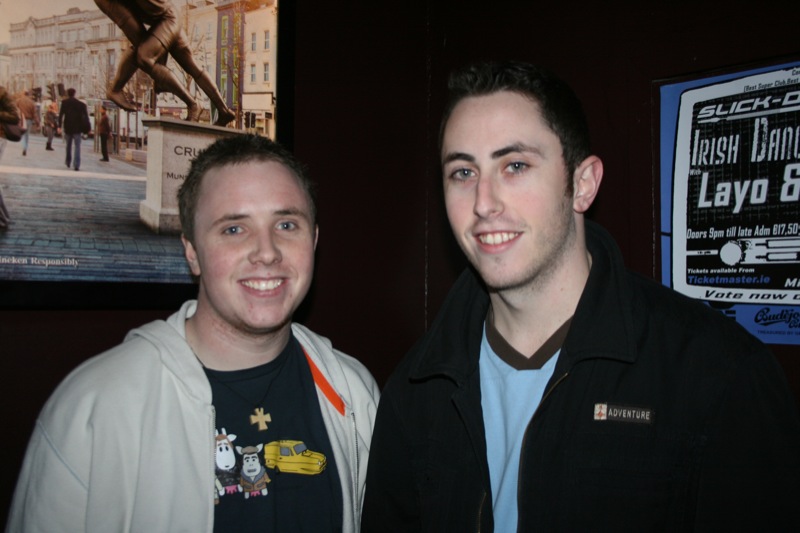The photograph is a detailed, color, indoor image taken in landscape orientation. It features two young men standing side-by-side, smiling warmly at the camera. Both men have blue eyes and short brown hair, with the taller man positioned on the right. The taller man, who has darker brown hair, is wearing a black jacket that says "adventure," paired with a blue t-shirt that has a brown collar neckline. The shorter man, standing to the left, has lighter brown hair and is dressed in a white zip-up hoodie over a black graphic shirt depicting cows and a yellow taxi cab. He also sports a wooden cross necklace. Behind them are several colorful posters mounted on the wall; one shows a cityscape with a statue in the foreground, while another features typography that partly reads "Irish." The scene captures a moment of camaraderie amidst a setting rich with visual detail.